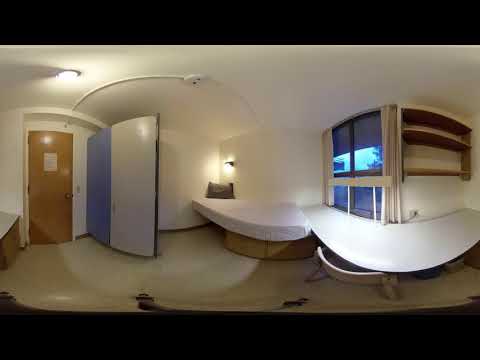This panoramic image captures an empty apartment or flat, likely staged for prospective renters or buyers. On the left, a wooden door with a white 8x10 piece of paper affixed to its upper half stands prominently, reflecting light above the paper. The walls are painted white, complementing the light beige-colored floor. At the center right, an intriguing modern bed, shaped like a half-circle cut in half, stands out. A pillow rests atop this unique bed, which features storage shelves underneath, adding to its functional design. Adjacent to the bed on the right is a curved, built-in table or desktop with wooden storage shelves above it. A window next to this setup offers a twilight view outside. The right section also features white objects, including a square one and a U-shaped one, both likely made of wood. Recessed lighting is embedded in both the ceiling and one of the walls, enhancing the room's ambiance.